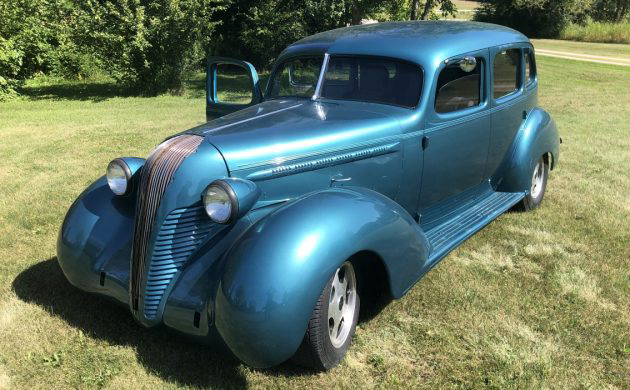This outdoor photograph showcases a classic, electric blue buggy car with considerable vintage charm. The car's front end is notably elongated, featuring a nose that's partially accented in gold or brown. It boasts a compact, square-shaped body with large, curved metal edges surrounding its sizeable black tires, which are contrasted by gray hubcaps. The hood of the car is distinctive with a triangular shape, bifurcated to display two small, centrally located headlights. The left door is open, while the right window is wound down, revealing a glimpse of the car's interior. Parked on a field of soft, short green grass, the car casts a shadow toward the bottom left of the image. The background also includes bushes and bright green trees, with a visible path or road in the top right corner of the photograph.